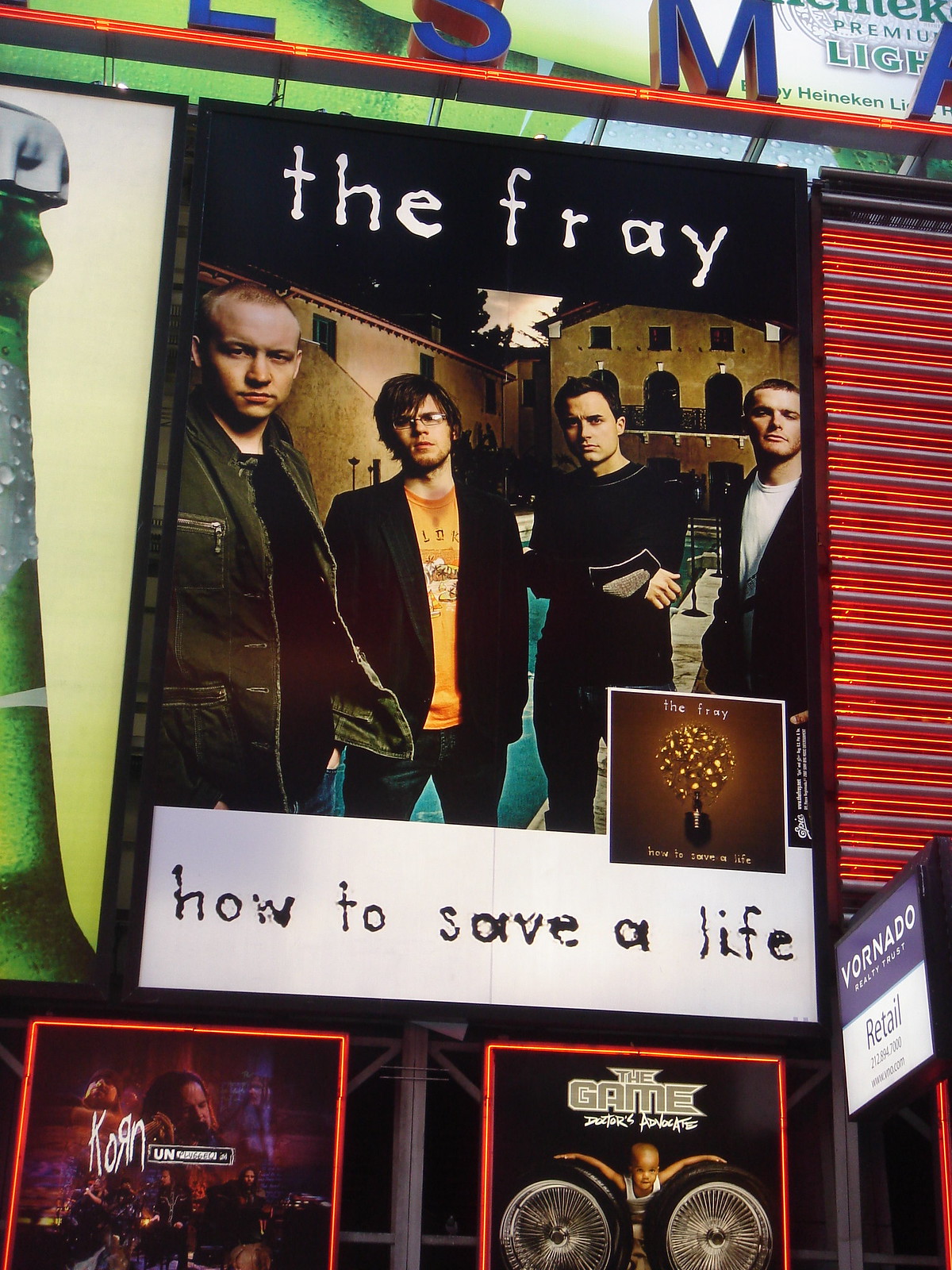The image showcases a large billboard or advertisement affixed to the exterior wall of a building. Dominating the top portion is an ad for the band The Fray, featuring the text "The Fray" in white against a black background. Below the band's name, the phrase "How to Save a Life" is displayed. The central part of the ad showcases four band members dressed in casual, predominantly black attire, gazing directly at the camera with somewhat stern expressions. They stand before a backdrop resembling adobe buildings, exuding a slightly grungy, urban vibe.

Beneath this main advertisement, two smaller posters are partially visible. The one on the left is for the band Korn, with the name stylized as "KORN" with the 'R' written backward. The poster on the right is for the rapper The Game. Both of these posters have a dark color palette, similar to the main advertisement above them. Additionally, there's a Heineken ad located in the upper right corner of the billboard setup, and another smaller ad with a black background and white text promoting Vornado Retail. The overall setting appears to be in front of a retail store, possibly indicating these albums are available for purchase inside.